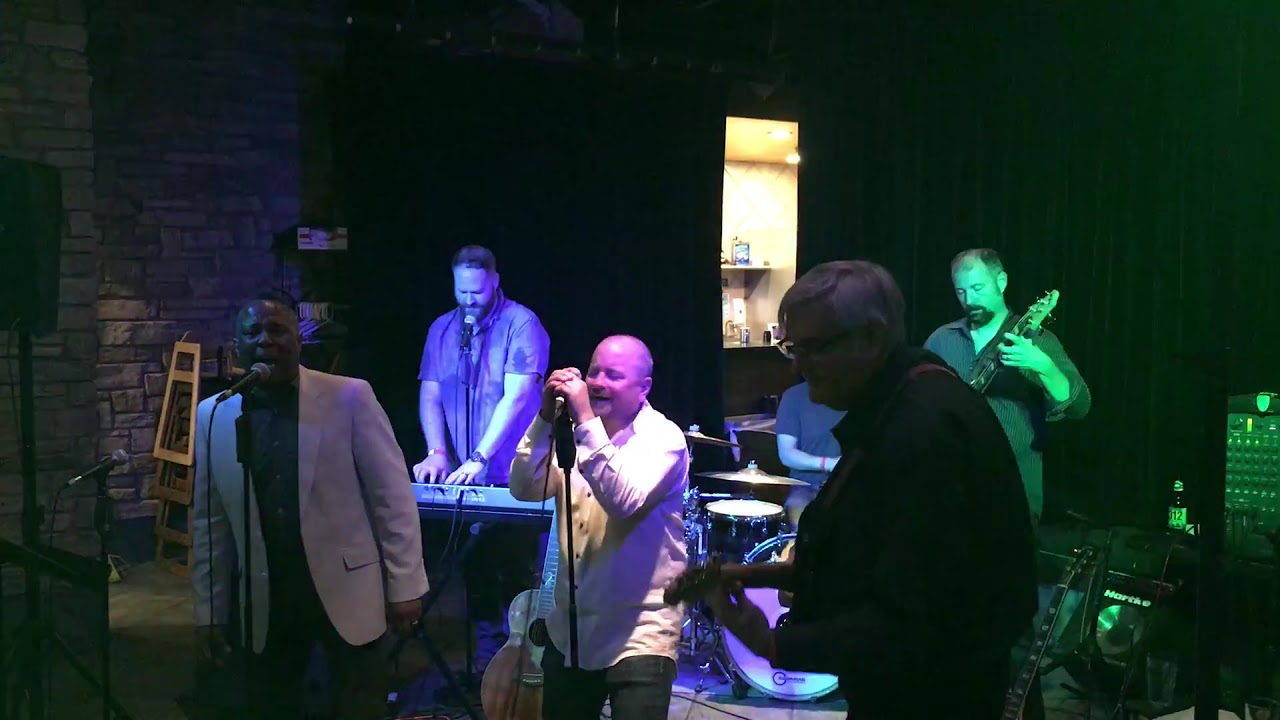The image depicts a band of six men performing on a dimly lit stage. At the front of the stage, two men are singing into a shared standing microphone. The first vocalist, a Black man in a blue shirt and white jacket, sings without holding the mic, while the second vocalist, a bald white man in a white shirt, holds the microphone as he sings. To their right, a man with white hair and glasses plays a guitar. Behind him, a man with a French beard also strums a guitar, with a green spotlight illuminating him. On the left side of the stage, another band member plays an electronic piano under a purple spotlight, and a microphone is positioned near his mouth, suggesting he may be singing as well. Further back, partially obscured, a musician plays a set of drums. The backdrop of the stage is predominantly dark, featuring a bright rectangular shelf at the far back, displaying various items and creating a contrast with the dim surroundings. The image also includes accent lighting in black, green, blue, pink, tan, and gray tones, with a distinct white spotlight highlighting the lead singer in the white shirt.